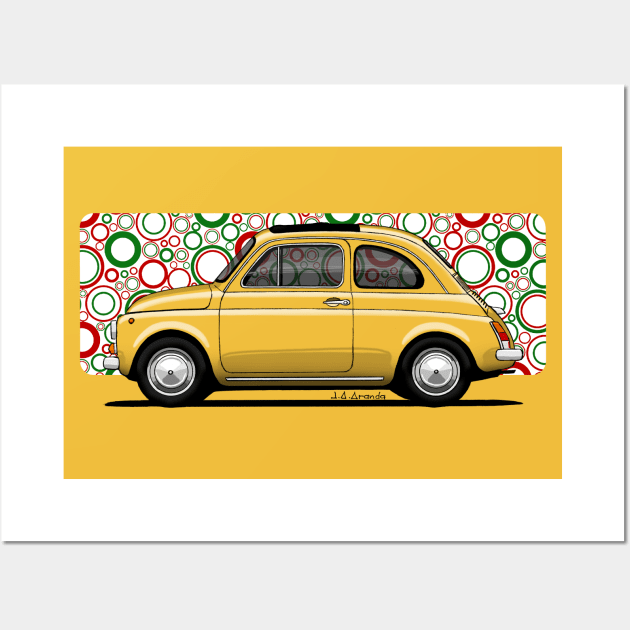The image is a vibrant art print with a distinct 1970s retro vibe, all set within a clean white frame against a light gray background. Central to the composition is a mustard-yellow rectangular box, inside of which lies another, more colorful rectangle. This inner rectangle bursts with a lively pattern of overlapping circles in various sizes and hues – greens, reds, blues, and oranges – reminiscent of a spirograph or mod artwork from the 1960s.

Dominating the scene is a sleek, vintage yellow hatchback car, akin to a 1960s Fiat 500, facing towards the right. The car features dark tinted windows, a single door, and a distinctive slanted hatchback, complete with a retractable sunroof and smooth black wheels. Below the car, a shadow grounds it in the space, and next to the rear wheel, the artist's signature, possibly "J.A. Aranda," is distinctly marked.

This intricate blend of textures and colors creates a nostalgic, yet dynamic visual experience, highlighting both the playful circular motifs and the streamlined elegance of the classic car.